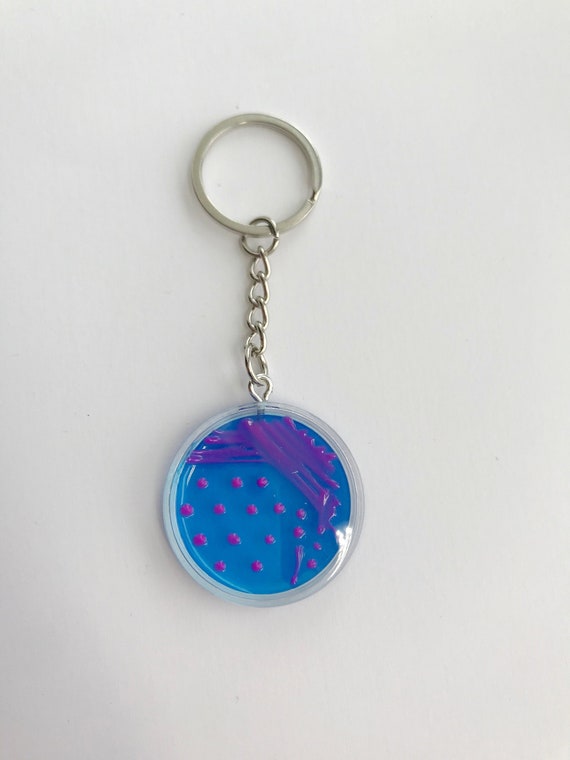The image features a keychain on a completely white background. The keychain consists of a standard silver circular ring attached to a link chain with six chain links. The decorative part of the keychain is a sizable circular medallion made of blue resin, which is semi-transparent, allowing some visibility through the blue. The outermost rim of the medallion is clear. Embedded within the blue resin are fluorescent pink dots and lines, with approximately fifteen pink dots scattered across the surface. The pink lines intersect and overlap, creating a visually dynamic pattern. The medallion has a slightly shiny appearance, indicating a plastic-like material. There are no shadows, emphasizing the keychain's presence on the stark white background.